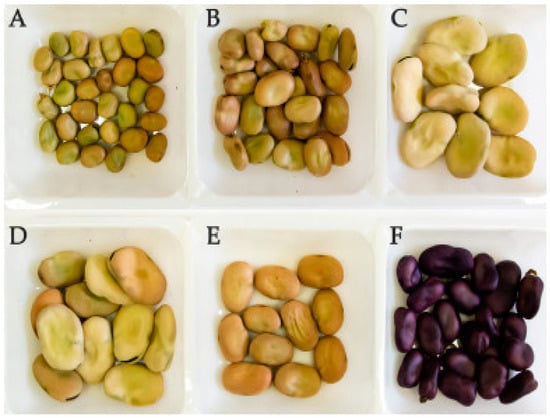This photograph showcases an organized array of six different types of beans or seeds, each displayed in shallow white dishes arranged in two rows of three against a plain white background. Each dish is labeled in the top left corner with black letters from A to F, proceeding left to right and top to bottom. 

Dish A contains small green and yellow seeds or beans, resembling young seeds or even popcorn kernels. Dish B holds a slightly larger variety of beans with a similar green and yellow color scheme, appearing somewhat like a mix of pistachios and peanuts. Dish C features a smaller quantity of very large, pale yellow to green beans, notable for their nearly white appearance with hints of green, resembling hazelnuts. Dish D also contains these pale, large beans, but in greater quantity and some appear to be cracking open slightly, giving them a unique texture reminiscent of banana chips. Dish E includes smaller, toasted brown beans that are darker, not cracked open, and scattered more abundantly. Finally, dish F displays deep purple beans with streaks of black or completely black beans, potentially resembling coffee beans or black beans. Each compartment reveals a hint of shine from the lighting, adding a subtle sheen to the presentation.